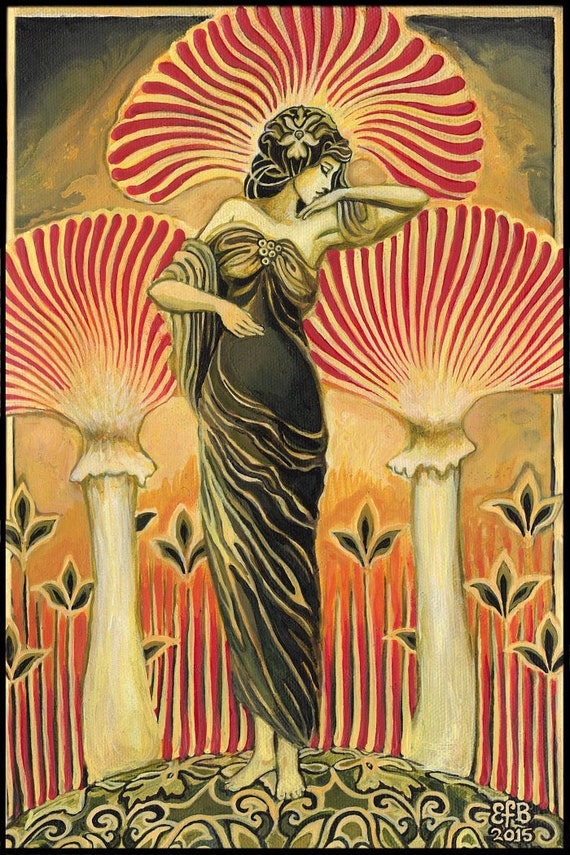A captivating image depicts a woman with long brown hair adorned with a flower, standing gracefully against a backdrop that resembles a vintage painting. She wears an elegant, strapless black gown that reaches the floor, characterized by a marbled pattern and subtle decorative circles along the chest area. The woman is leaning slightly on her left hand, which is raised to shoulder level with her palm facing down, while her right arm is bent at a 90-degree angle, also with the palm facing down. Surrounding her are three enormous mushrooms, their white stems juxtaposed with vibrant red gills that form shell-like shapes. These mushrooms, as tall as the woman herself, add a whimsical and surreal touch to the scene. The background features a blend of orange and black hues in the upper corners, all enclosed by a thin black border and a light yellow or tan inner border, enhancing the overall vintage poster feel. The woman stands on a green, round platform adorned with intricate designs, completing the enchanting scene.